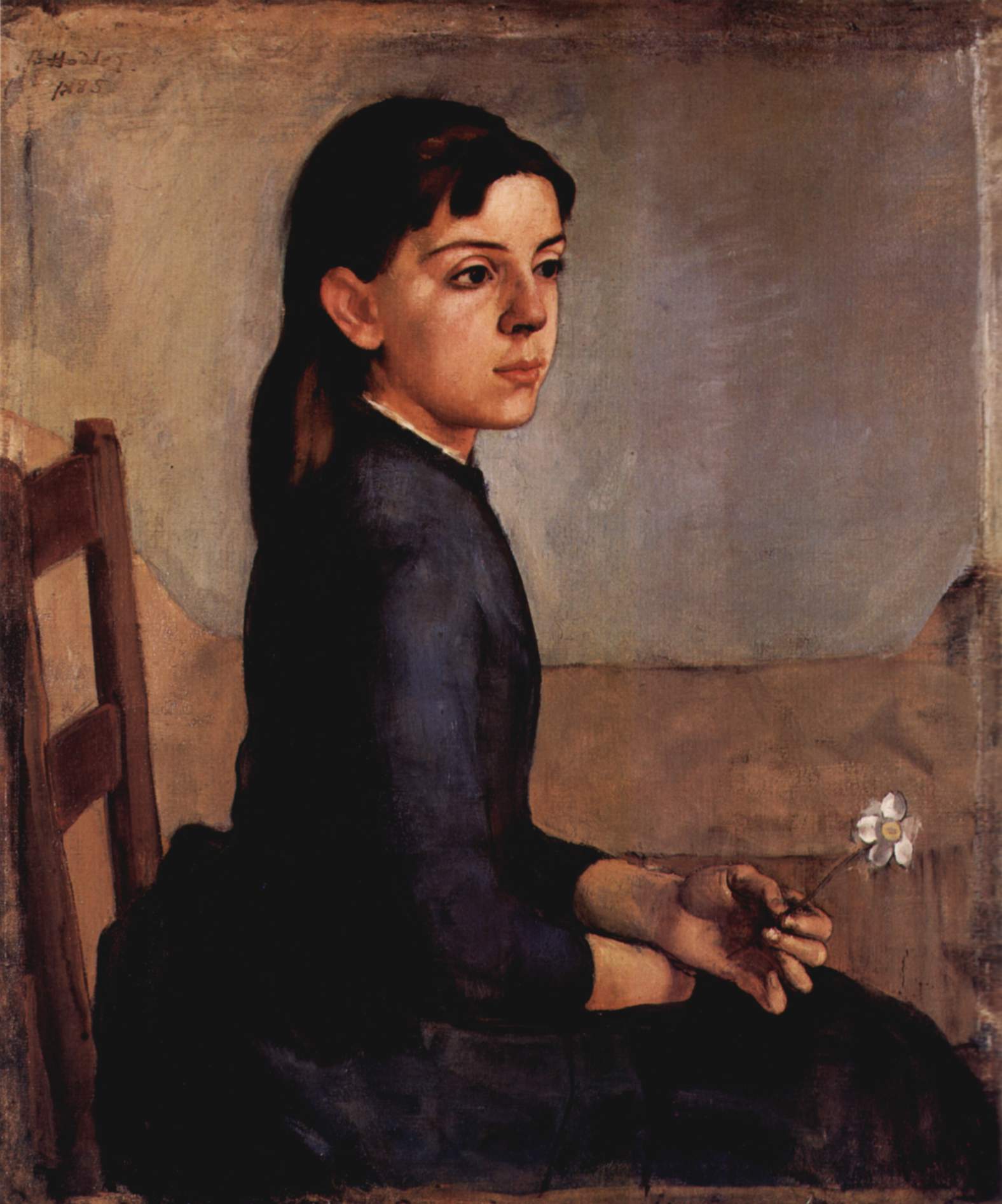The watercolor painting portrays a young girl seated on a simple brown wooden chair with two vertical supports on the backrest. She is depicted in a three-quarter view, seated towards the left while gazing slightly to the right. The girl has dark brown hair parted down the middle, with strands gently touching her forehead on either side, and the rest cascading down her back. Her hair reveals her ears completely. She has light skin, dark brown eyes, and pink lips, with a subtle shadow adding depth to the right side of her face.

The girl is dressed in a heavy blue dress with long sleeves that nearly reach her wrists. The dress's plush fabric creates a slight bulge at the small of her back. Both of her hands and wrists appear slightly dirty, with her left hand delicately folded over her right. She holds a daisy with white petals between her index and pinky fingers of her left hand. The background features a neutral palette of grays, light browns, tans, and off-whites, softly blending to provide a muted, complementary backdrop to her figure. The painting is vertical, taller than it is wide, enhancing the portrait focus on the young girl.